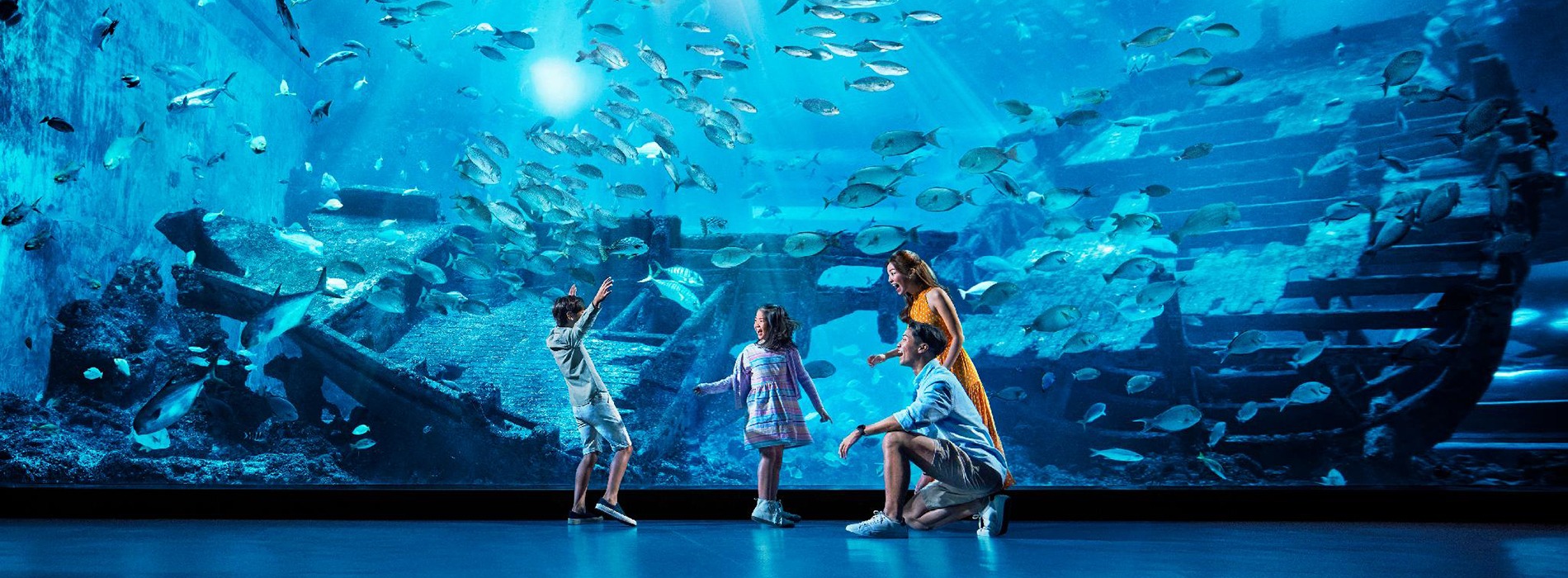A vibrant photograph captures a delighted family of four posing in front of a large glass aquarium tank filled with various small fish and a sunken ship decoration. The aquarium scene includes a blue reflective floor and the image focuses on the family, suggesting a happy, possibly orchestrated, moment. Central in the frame is a little girl with dark long hair, dressed in a white dress adorned with three blue horizontal stripes and royal blue shoes. Beside her, slightly to the left, a young boy energetically raises his arms diagonally. He is dressed in a green shirt and blue shorts, paired with dark shoes featuring white bottoms. To the right, the mother stands in an eye-catching orange dress, her long brown hair cascading down. Partially in front of her, the father kneels, wearing a blue shirt with rolled-up sleeves, gray shorts, and shoes that appear white or blue. The family appears engaged and pleased, sharing in the exuberance of the aquarium experience, with both parents and the sister smiling warmly at the lively gestures of the young boy. The backdrop features many fish, slightly indistinct due to the resolution, swimming around the remnants of what looks like a sunken pirate ship, adding an adventurous touch to the serene underwater scene.